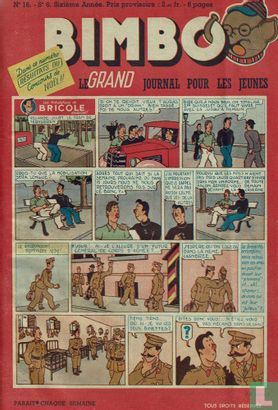This image features a retro comic book page set against a red background, displaying slightly faded colors typical of older comics or newspaper clippings. The top of the page prominently reads "Bimbo" in white, three-dimensional block letters, with the phrase "Le Grand Journal pour la Jeunesse" beneath it, indicating it is a French-language comic aimed at young readers. A humorous cartoon elephant head, donning glasses and a small hat with its tongue playfully sticking out, is positioned in the upper right corner, with its trunk threading through the O in "Bimbo" and appearing to support it.

The comic strip itself is divided into multiple panels arranged in a grid format. The panels feature small, illegible speech bubbles and portray various scenes. The top half focuses on outdoor scenes with a number of characters, while the lower half depicts figures in military uniforms—tan and olive garb—engaged in conversation. The lower right corner includes some additional French text starting with a large letter "L." Overall, the image reflects the nostalgic charm of vintage comics with its detailed artwork and storytelling.